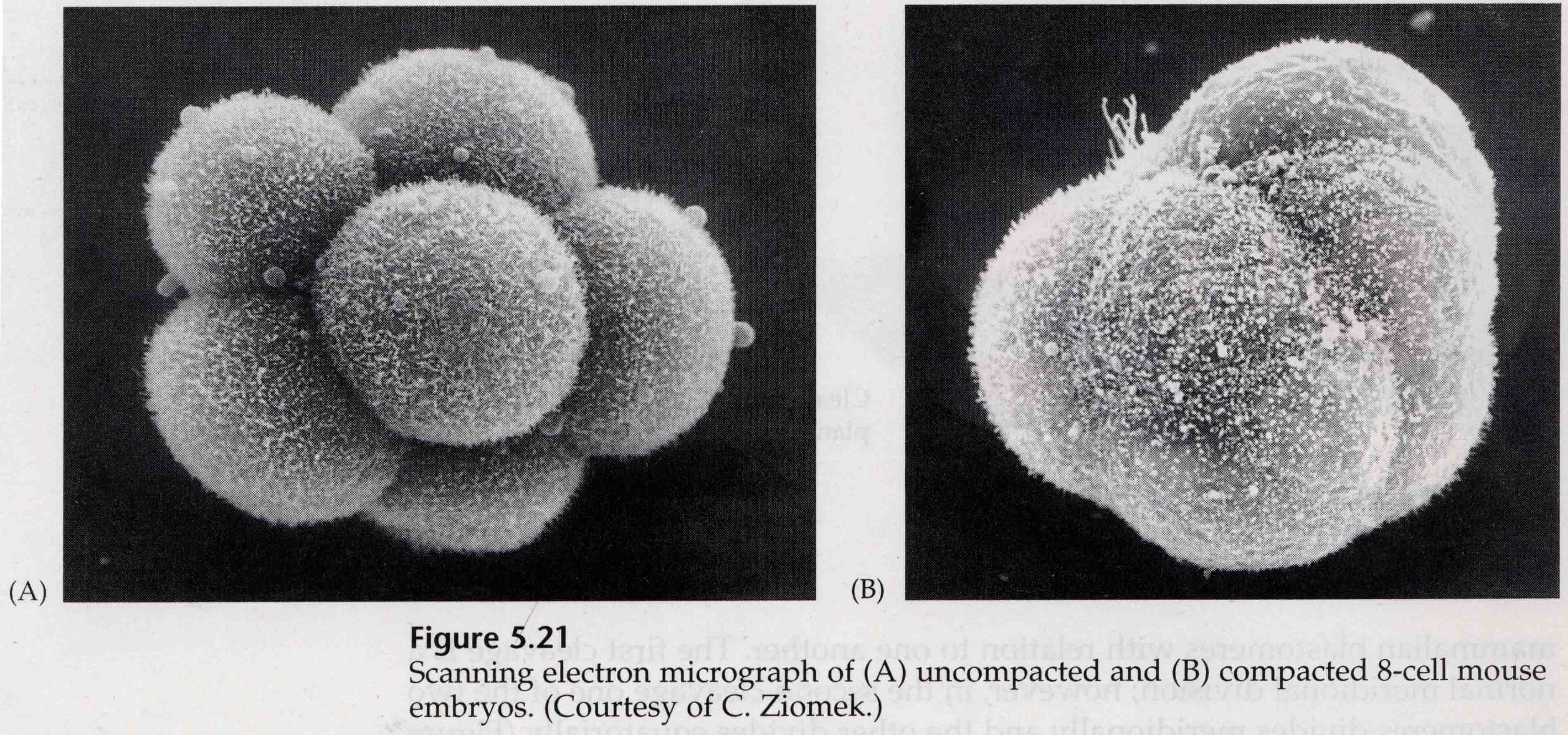The image, seemingly scanned from a textbook, features two highly magnified black-and-white photographs of mouse embryos labeled "A" and "B". The photograph on the left, marked "A", displays five round, fuzzy spheres representing uncompacted eight-cell mouse embryos. The photograph on the right, labeled "B", shows a single compact mass of these spheres, depicting the compacted state of eight-cell mouse embryos. The page appears to be part of a book, as faint text from the other side is visible. Below the images, the caption reads: "Figure 5.21: Scanning electron micrograph of A) uncompacted and B) compacted eight-cell mouse embryos (Courtesy of C. Zeomech)".